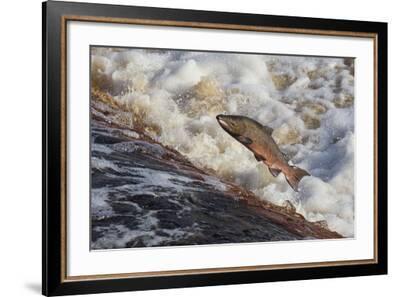The image depicts a photograph of a dark green and brown salmon with a pinkish belly, mid-leap out of turbulent, dirty water, likely in an attempt to swim upstream over a waterfall. The water appears frothy and crashing, suggesting dangerous rapids. The photograph is displayed within a sophisticated picture frame consisting of a black outer border, an inner gold rim, and a protective white matte surrounding the image. The frame is tilted slightly to the right, creating a subtle shadow behind it, emphasizing the three-dimensional presentation of the art piece. The composition highlights the salmon's struggle and the dynamic movement of the river.